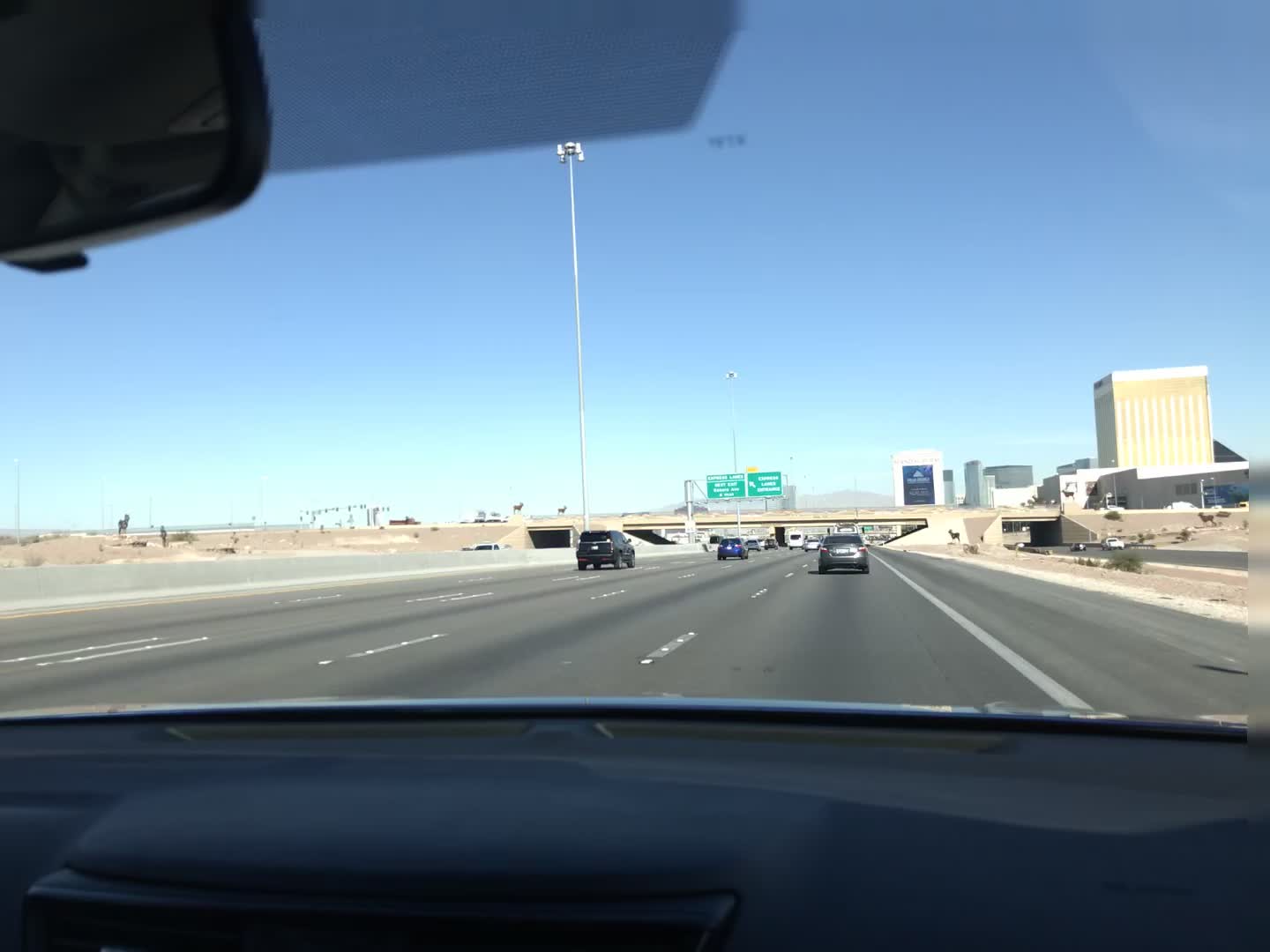This photograph captures a moment on a vast interstate, where the scene is divided by contrasting elements on either side. On the left, the landscape is barren and appears desolate, devoid of any significant features. In stark contrast, towering on the right is an impressive skyscraper hotel, serving as a prominent landmark against the otherwise flat horizon.

The interstate itself is a busy thoroughfare, with four lanes dedicated to vehicles traveling in the same direction. Positioned on the far right side of the highway, the shoulder is clearly visible, creating a buffer between the fast-moving traffic and the skyscraper.

Ahead, green wayfinding signs indicate upcoming exits and destinations, helping drivers navigate their routes. The roadway is busy with various vehicles including a small white bus, an SUV, and several other cars scattered along the lanes.

The sky above is a clear, vibrant blue, adding a sense of openness to the scene. On the left side of the image, there seems to be either a cactus or a donkey, though it is difficult to distinguish with certainty.

Adding another layer of interest to the composition, a bridge looms in the distance, which the road will pass under shortly, integrating elements of architecture and transportation infrastructure into the landscape.